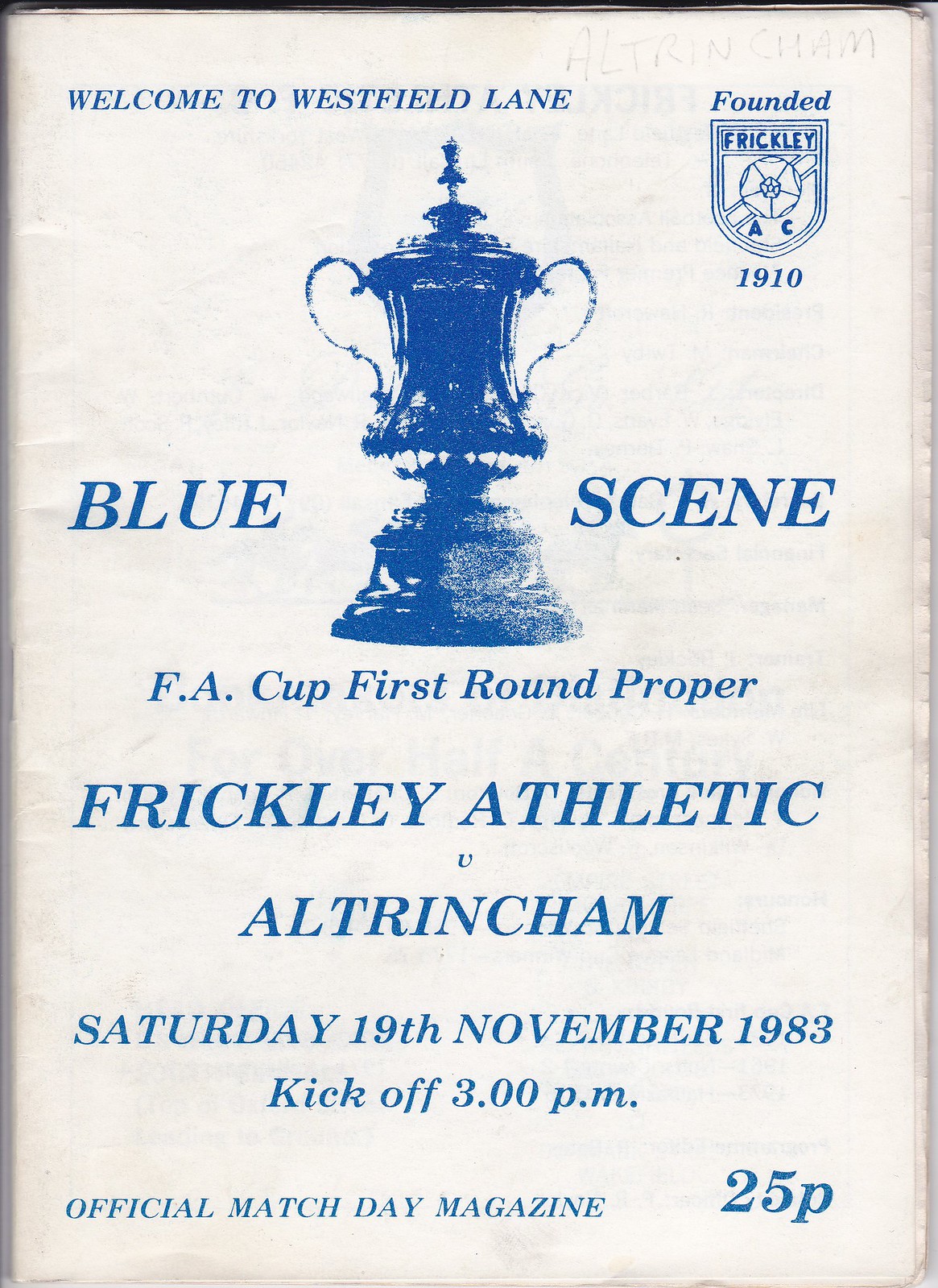The front cover of the soccer program is an old-timey design dominated by blue and white colors, with a simplistic white background and all the lettering and logos rendered in blue ink. At the top left corner, the text "Welcome to Westfield Lane" is prominently displayed. In the top right corner, there is a logo featuring a shield with a soccer ball, accompanied by the text "Founded Frickley A.C." and the year "1910."

At the center of the cover, an ornate award trophy captures immediate attention. Flanking the trophy on either side are the words "Blue Scene." Below this, in smaller letters, it reads "FA Cup First Round Proper," followed by "Frickley Athletic" on the next line, a small "V," and then "Altrincham" (spelled A-L-T-R-I-N-C-H-A-M).

Further details underneath include the match date, "Saturday, 19th November, 1983," and the kickoff time, "3 o'clock p.m." Along the bottom edge of the program, the phrases "Official Match Day Magazine" and "25p" are printed in smaller font, providing additional information about the publication.